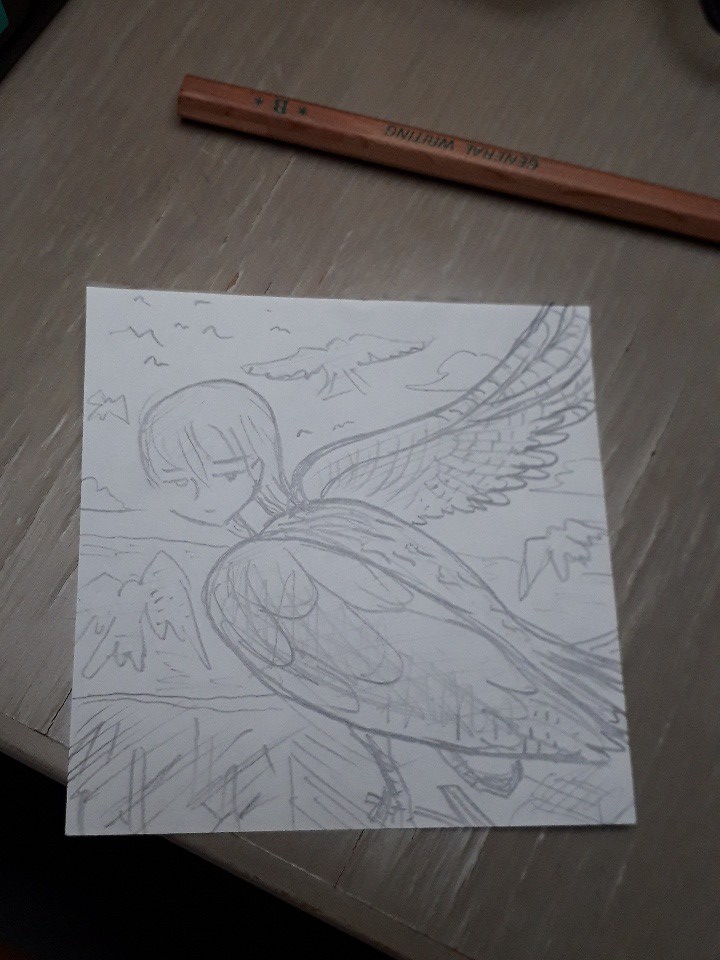The image depicts a detailed pencil drawing on a piece of white paper, which rests atop a grainy, gray-painted wooden table. The central figure of the drawing is a bird with its body shown in profile. Notably, one of its wings is extended outwards, displaying intricately detailed feathers, while the rest of its body remains still. The bird's head is artistically replaced by the head of a young girl, turned sideways in a manner that gives the impression she is glancing over her shoulder. Surrounding the primary figure, the sky is populated with several other birds, each with their wings spread wide in flight, along with a scattering of clouds that add depth to the scene.